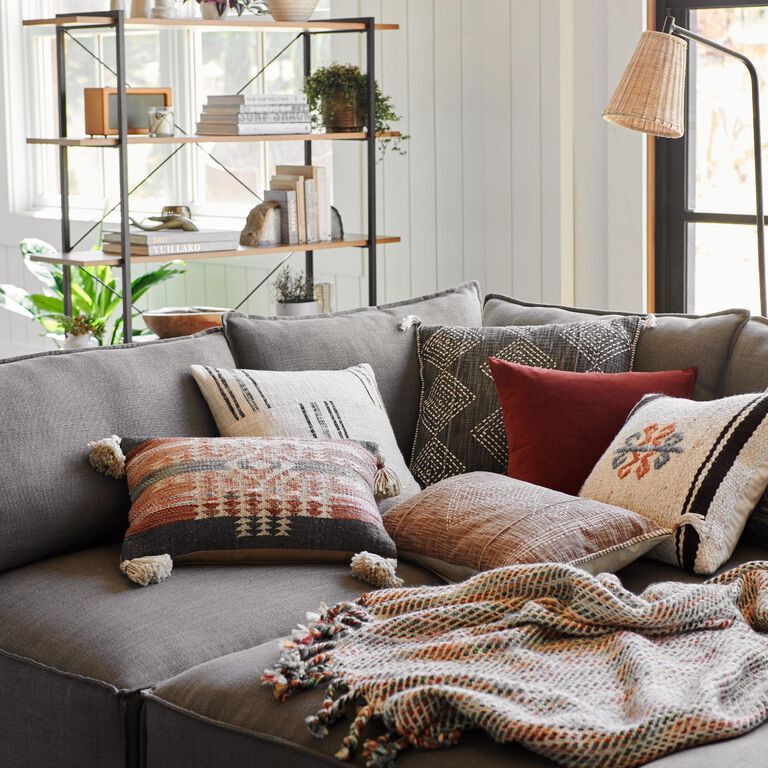The photograph depicts a cozy, inviting living room centered around a gray sectional sofa accented with six throw pillows of various black and white, red and white patterns, and some with embroidery. The pillows feature natural fabrics with rustic, heavy weaves and white tassels at the corners. A woven coral and gray throw blanket is casually draped across the sofa, adding to the comfortable ambiance. The backdrop includes vertical white wood paneling and a floor lamp with a tan straw shade positioned for reading. Natural light streams through two large windows, one partially concealed by a rubber plant in a large pot. To the left, a minimalist metal-framed bookshelf with wooden shelves houses books, small plants, a radio, pottery, and decorative objects, contributing to the room's relaxed, Southwestern style. The overall setting is bright and airy, evoking the charm and warmth of a pottery barn catalog scene.